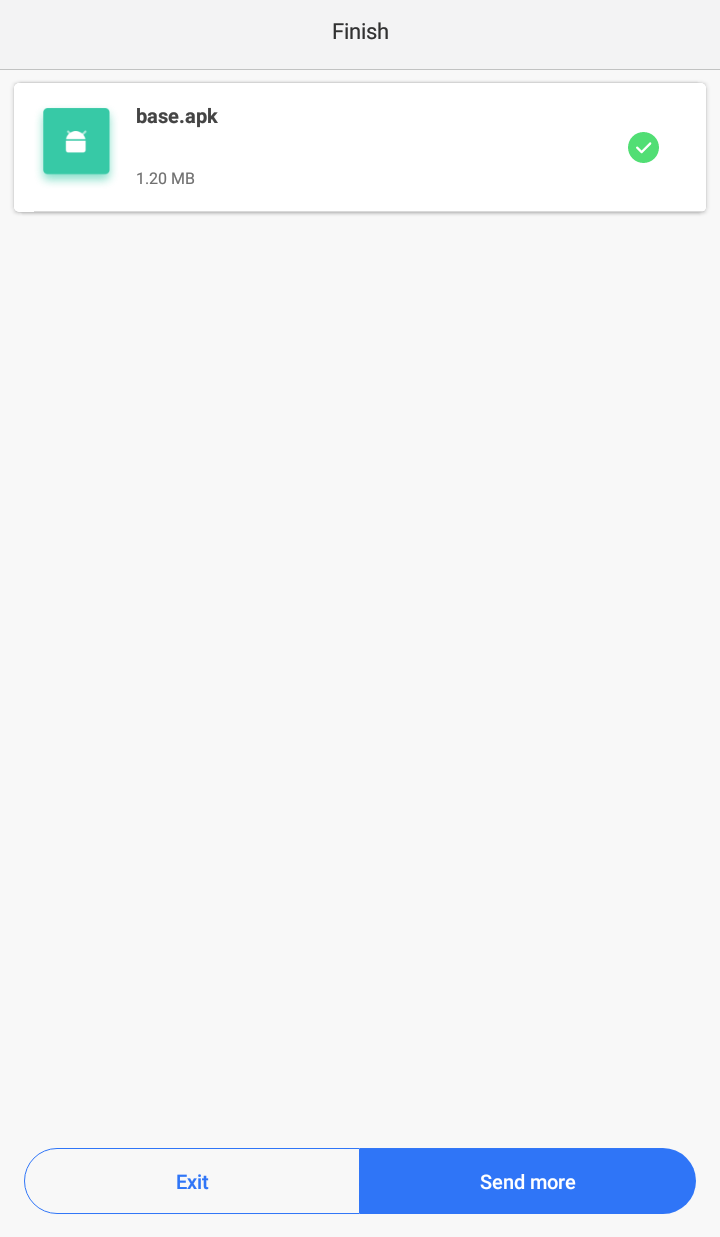This image is a cropped mobile screenshot depicting the installation of a base APK file. At the top center, there is the word "Finish" in a small, bold black font. Below this, a large white rectangle dominates the screen, featuring a green square icon with an Android figure on the left. Next to the icon, the text "base.apk" is displayed in bold, lowercase letters. Underneath this, "1.20 megabytes" appears in small, gray font, and to the far right of the rectangle is a green circle icon containing a white checkmark. The rest of the page is blank, except for the bottom section that houses two buttons. The button on the left, outlined in blue, reads "Exit" in the center with bold blue font. The button to the right, labeled "Send More," is highlighted in blue, indicating it is currently selected.